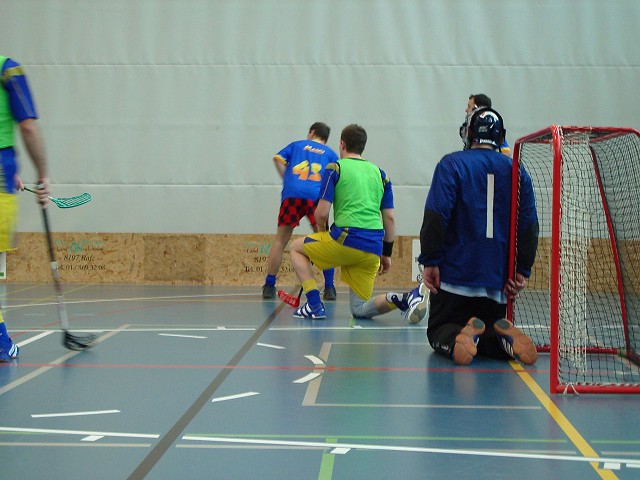This photo captures a dynamic moment in an indoor floorball game, set in a gymnasium with white fabric walls featuring vertical sewing lines, and a plywood base marked with stamps and logos. The blue floor is detailed with a yellow line by the goal, a small white box in front of the goal, and a dashed circle directly behind the box. 

The goalie is on his knees in the net, wearing a black helmet and a long-sleeve blue shirt with the number one on the back. His orange shoes have a distinct black circle on the heel. The net behind him is red with white netting. Centered in the frame, a player in a green vest, blue shirt, and yellow shorts is kneeling down, while another player on the left, partially visible, holds a floorball stick and also wears a green vest and blue sleeves. 

In the far distance, a player sporting red checkered shorts looks to the left. The mismatched uniforms among the five visible players contrast sharply, highlighting the casual or mixed-team nature of the game. Everyone in the image is facing a different direction, adding to the sense of spontaneous action captured in this scene.